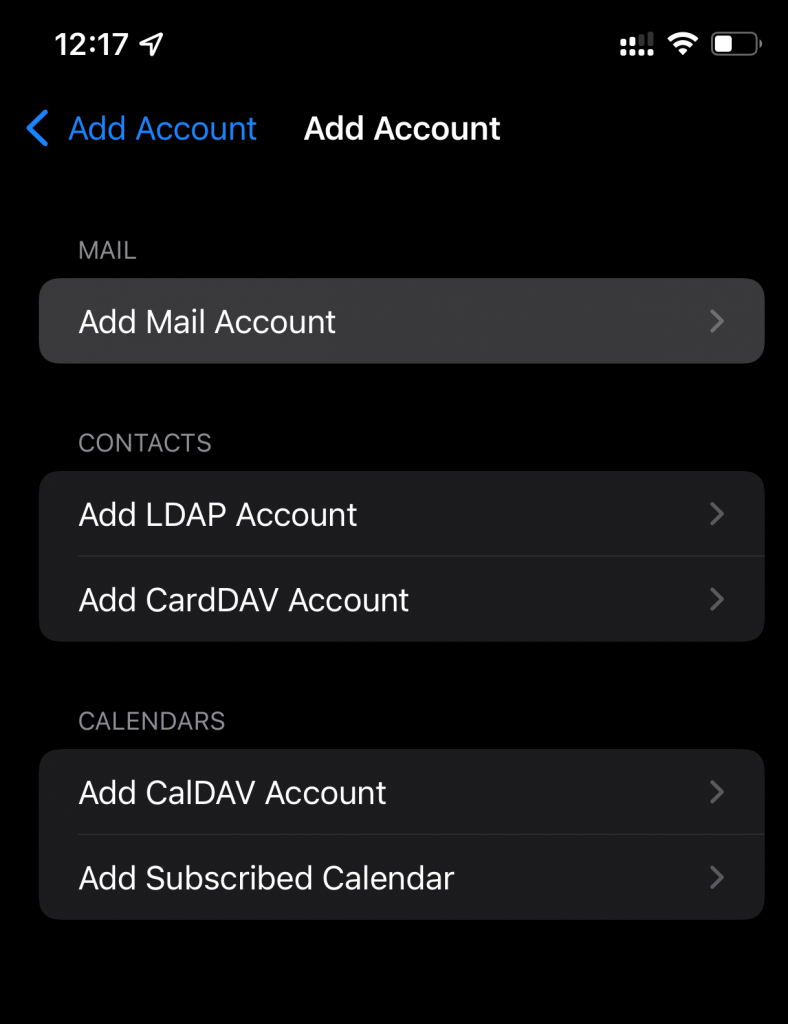The image is a screenshot from a smartphone with a black background. At the top left corner, the time is displayed as 12:17, though it doesn't specify whether it's a.m. or p.m. On the top right corner, there are several icons: a battery icon indicating about half charge, a Wi-Fi icon, and a wireless connection icon.

Below these icons, in the center header area, the text "Add Account" appears in white font. To the left of this, the same text "Add Account" is displayed in blue font, accompanied by a left-pointing arrow on the left side.

Further down, against the black background, the word "Mail" is shown in gray font on the right side. Beneath it, there is a large, dark gray rectangle with rounded corners that reads "Add Mail Account" in white font.

Proceeding below, the word "Contacts" appears in gray font, followed by another dark gray rectangle with rounded corners, labeled "Add LDAP Account" in white font. Directly beneath this, it says "Add CardDAV Account" in white font.

Continuing down, the word "Calendars" is displayed in gray font against the black background, followed by a dark gray rectangle with white font reading "Add CalDAV Account." Underneath, there is a white font text reading "Add Subscribed Calendar."

Each dark gray rectangle features a tiny right-pointing arrow on its right side.